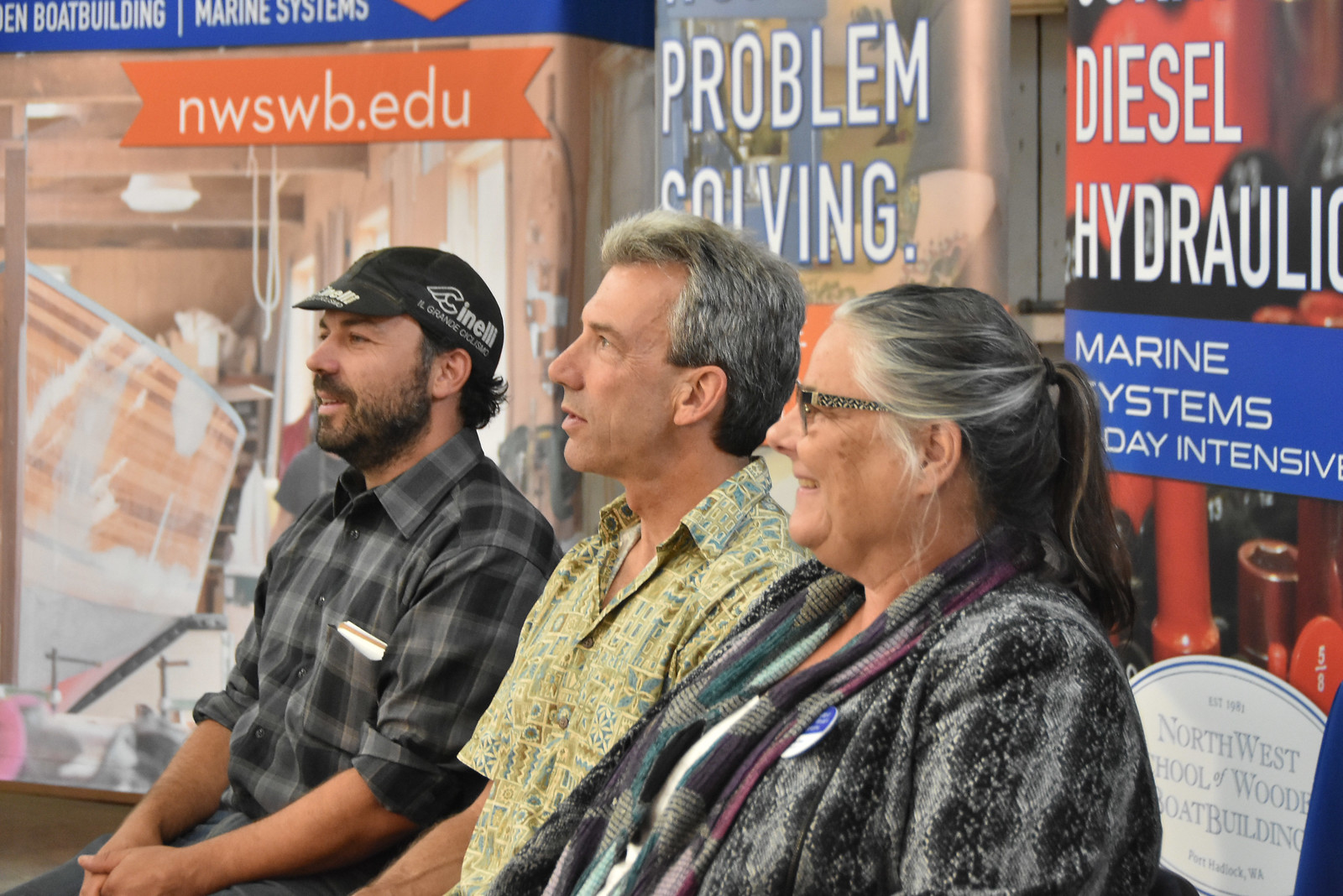This photograph captures three individuals seated next to each other on a bench in front of a building adorned with various advertisements. Positioned under banners that read "NWSWB.EDU," "Diesel Hydraulics," "Marine Systems," and "Problem Solving," the backdrop provides a technical or educational context, with displays indicating terms like "NAE Intensive."

On the far right, an elderly lady wears a black and gray coat, complemented by a scarf featuring purple and green designs. Her hair, a mix of gray and dark black, is mostly pulled back, with a small strand hanging just under her ear. She also wears eyeglasses and gazes directly to the left.

In the middle, a Caucasian man with short, frosty blonde hair that darkens at the back, sports a button-up shirt with green and blue colors. He sits slightly forward, seemingly engaged with the scene to his left.

To his left, another man in a black cap and full beard dons a plaid shirt with the sleeves rolled up. A white card sticks out from his pocket, and he rests his hands in front of him.

The group appears to be observing something of interest, their gazes collectively directed towards the left side of the frame, all while positioned in front of a wall full of informative displays.